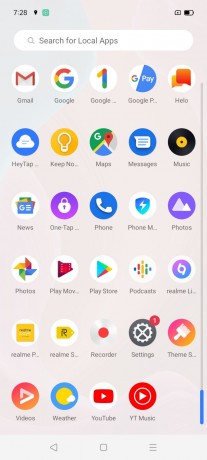This screenshot captures a smartphone interface featuring a detailed list of applications. The screenshot was taken at 7:28, as indicated by the displayed time. A location icon is visible, accompanied by a battery icon showing a 60% charge. Below this information is a search bar with the placeholder text "search for local apps," accompanied by a magnifying glass icon.

The first set of apps, listed in the top row, includes Gmail, Google, Google One, Google Pay, and an app named Halo (spelled H-E-L-O). The second row contains the following apps: Haytap, Key & O, Maps, Messages, and Music. 

Moving further down, the apps listed include News, OneTap, Phone, Phone M, and Photos. This is followed by Play Movie, Play Store, Podcast, Real Me, Real Me P, Real Me S, and Recorder. The Settings app, which has a red notification badge with the number one, is listed next. Lastly, the list includes Themes, Videos, Weather, YouTube, and YT Music apps.

Each application is precisely arranged, providing an organized view of the phone's interface.